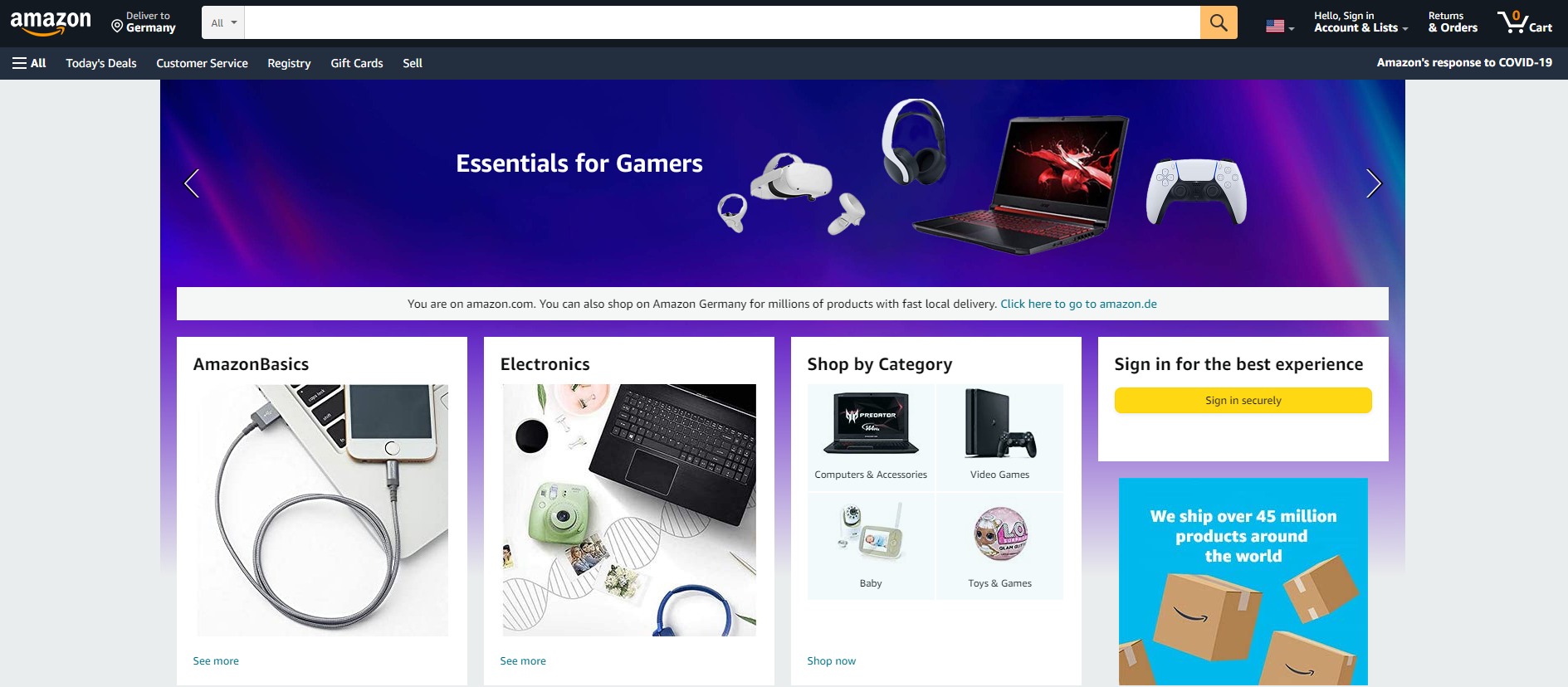Sure, here is a cleaned-up, detailed caption for the image described:

---

The image appears to be a screenshot of an Amazon webpage. On the top left, there is the Amazon logo featuring "Amazon" with an A to Z orange arrow. Below the logo, the text "Germany" is displayed. Adjacent to this, there is a search bar on the left side, accompanied by a yellow square with a magnifying glass icon. Towards the top right, the U.S. flag is present, alongside options that read, "Hello, Sign in," "Accounts and Lists," "Orders," and a shopping cart icon with a yellow circle inside it indicating item count.

Underneath the navigation bar, a menu showcases various categories including "Today's Deals," "Customer Service," "Registry," "Gift Cards," and "Self." The website seems to be promoting a special section titled "Essentials for Gamers," highlighted within a blue rectangle.

In the main section, gaming-related products are displayed, including an Oculus Quest headset with two controllers, a Pulse headset, and a laptop. Further down, products under the "Amazon Basics" label are shown, such as a laptop with a cable plugged into a phone, various electronic gadgets, an open laptop keyboard, and a digital camera. Additional items like a wavy DNA structure graphic, a Shopify category suggestion, a laptop, and PlayStation accessories are also visible.

Bars are seen on the left and right sides of the screen, framing the main content area.

---

This caption helps describe the layout and elements of the Amazon webpage in a detailed manner.